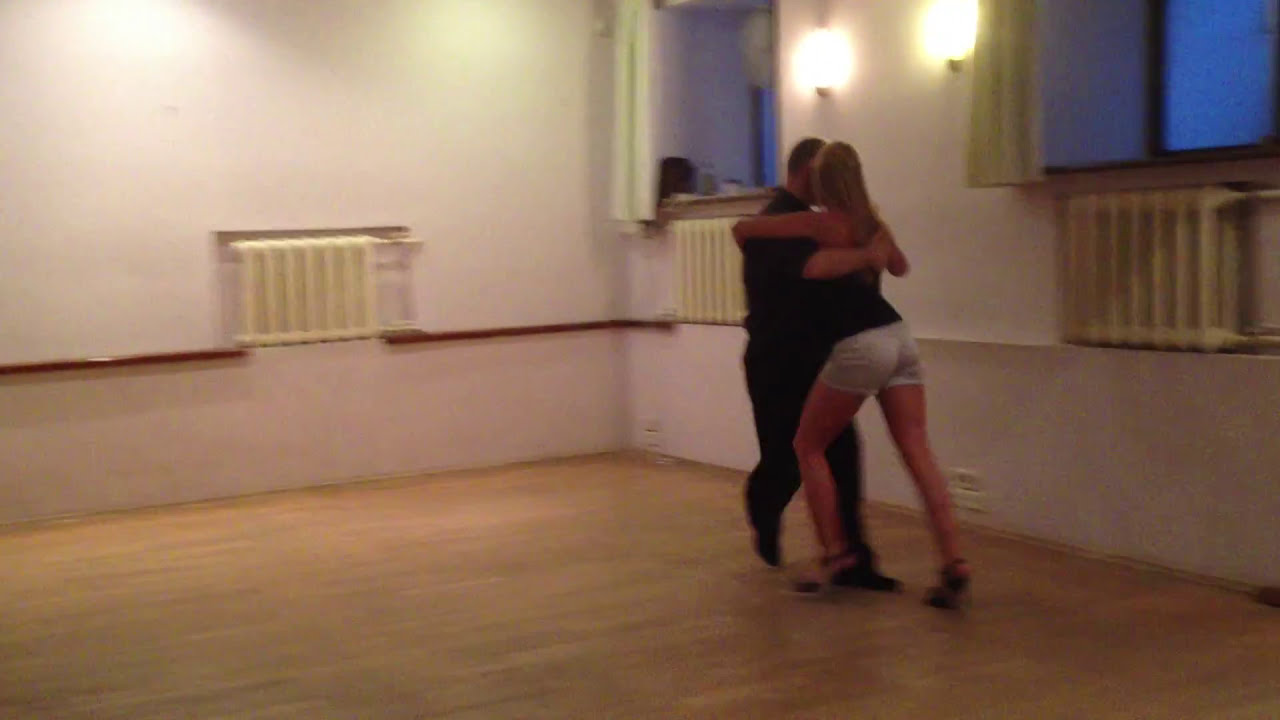In a slightly blurry image, two dancers are captured mid-movement in an indoor studio, framed on the right third of the composition under two wall sconce lights. The male dancer, dressed in all black, appears to be leaning backward, while the female dancer, with long mid-length blonde hair, sports a black tank top, light-colored shorts, and black high heels, leaning in towards him. They have their arms and upper bodies locked in a dynamic pose that hints at a flowing dance sequence. The spacious studio, characterized by its light cream walls and wooden floors, appears to be empty except for them. The walls feature apparatus and seem to have radiators or air conditioning units, with a brown rail running along the edge. Two large windows on the right-facing wall reveal a dusk or nighttime scene outside, adding to the romantic ambiance illuminated by the indoor lamps.